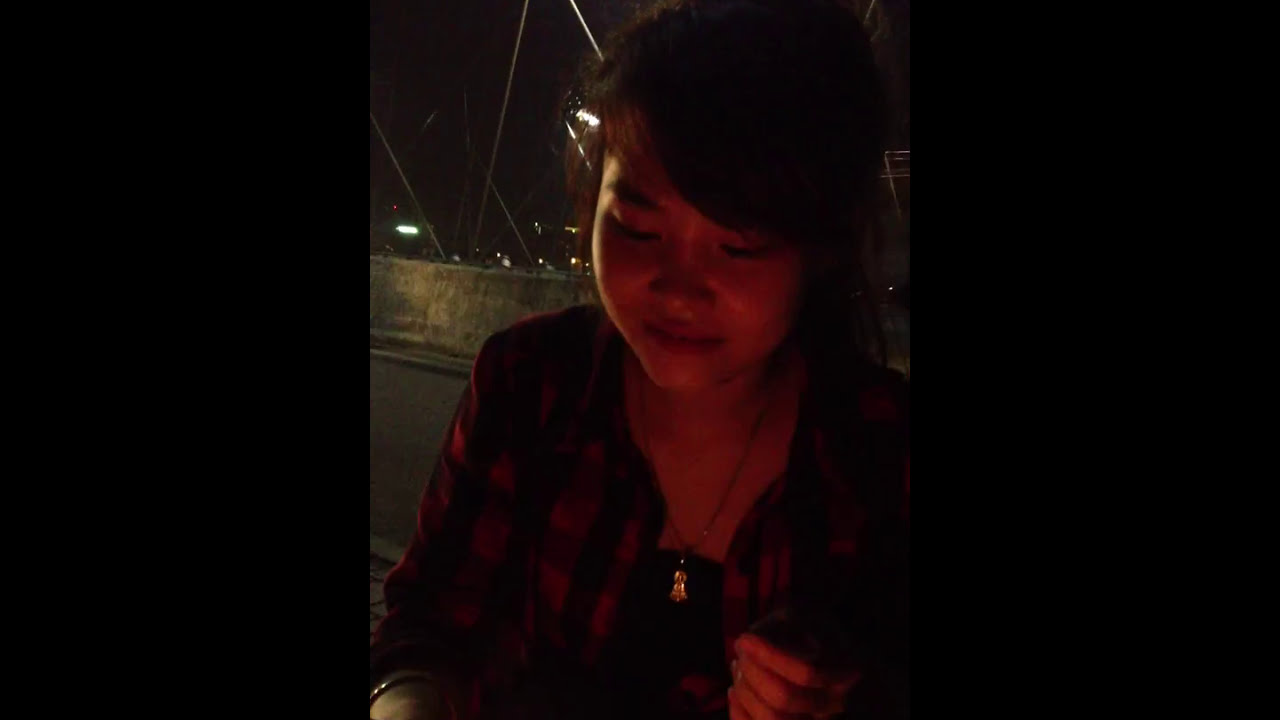The photograph captures a young woman of Asian descent with dark, long hair and a lighter skin complexion. She is adorned with a necklace featuring a pendant and multiple bracelets. Her attire includes a red and black checkered flannel jacket over a black undershirt. The young lady's eyes are focused downward, seemingly engrossed in something on her phone. 

She stands alone, illuminated by a red light that casts a glow on her face and upper body, adding a dramatic effect to the nighttime scene. The background reveals a cityscape with faint lights from buildings or homes and what appears to be a road or a sidewalk bordered by a small wall. The overall ambiance of the image is dark, yet the subject is clearly visible, making her the focal point of the photograph.